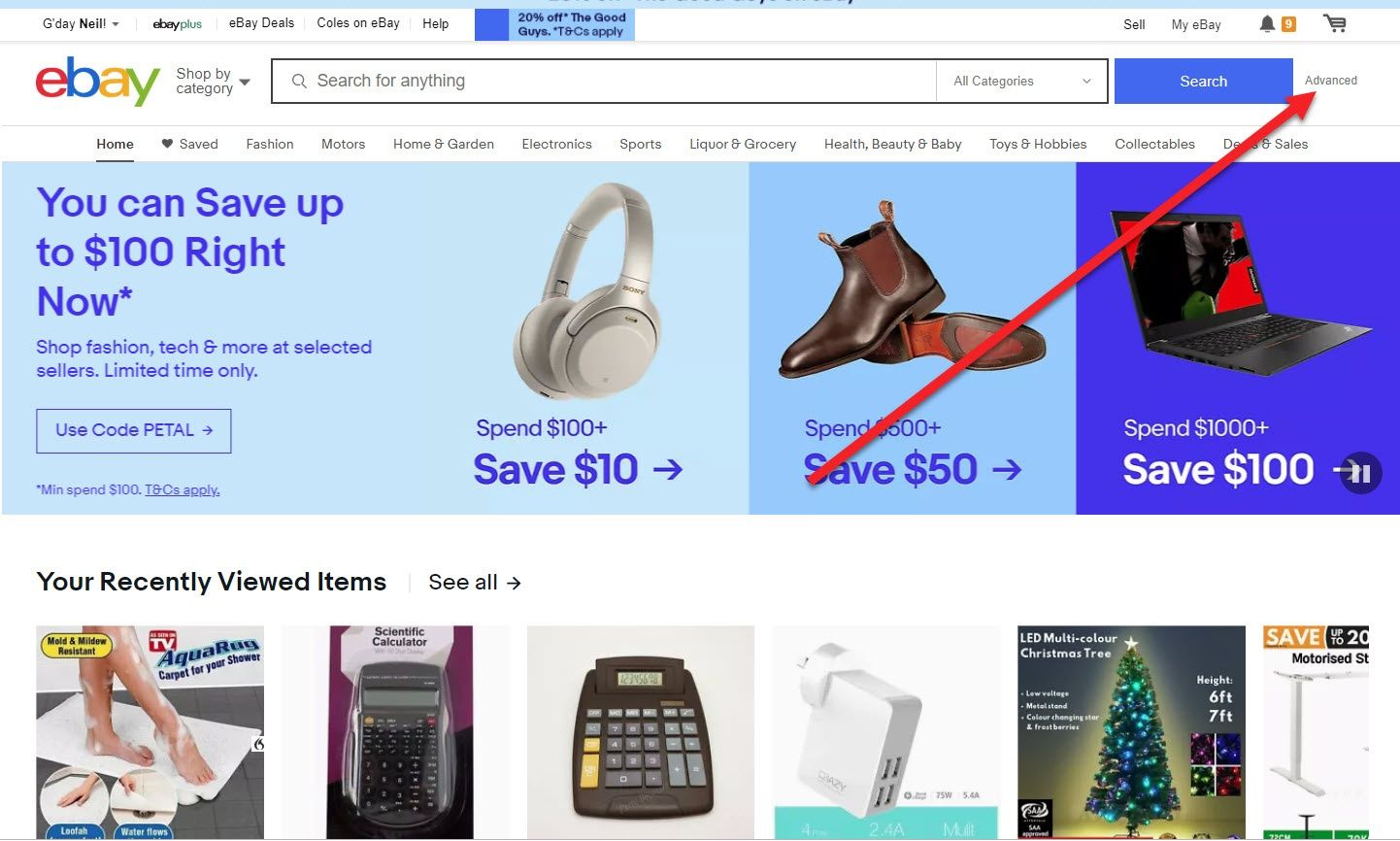A detailed screenshot of a user's computer screen displaying the eBay homepage. At the top, the familiar eBay search bar and subcategory navigation are prominently visible, showing categories such as Fashion, Motors, Home & Garden, Electronics, and Sports. Below the search bar is a large promotional banner offering savings of up to $100 with code "PEDAL." The banner features images of various electronic and fashion items including a pair of headphones and women's boots, with specific discount details: "$100+ spend, save $10" and "$500+ spend, save $50."

Further down, the screenshot shows a section highlighting the user's recently viewed items, displaying thumbnail images of a calculator, a Christmas tree, and a foot massager marked "As Seen on TV," among other products. The most striking element of this screenshot is a large red arrow superimposed on the homepage, pointing towards the "Advanced" link next to the search bar, indicating an emphasis on utilizing the advanced search functionality.